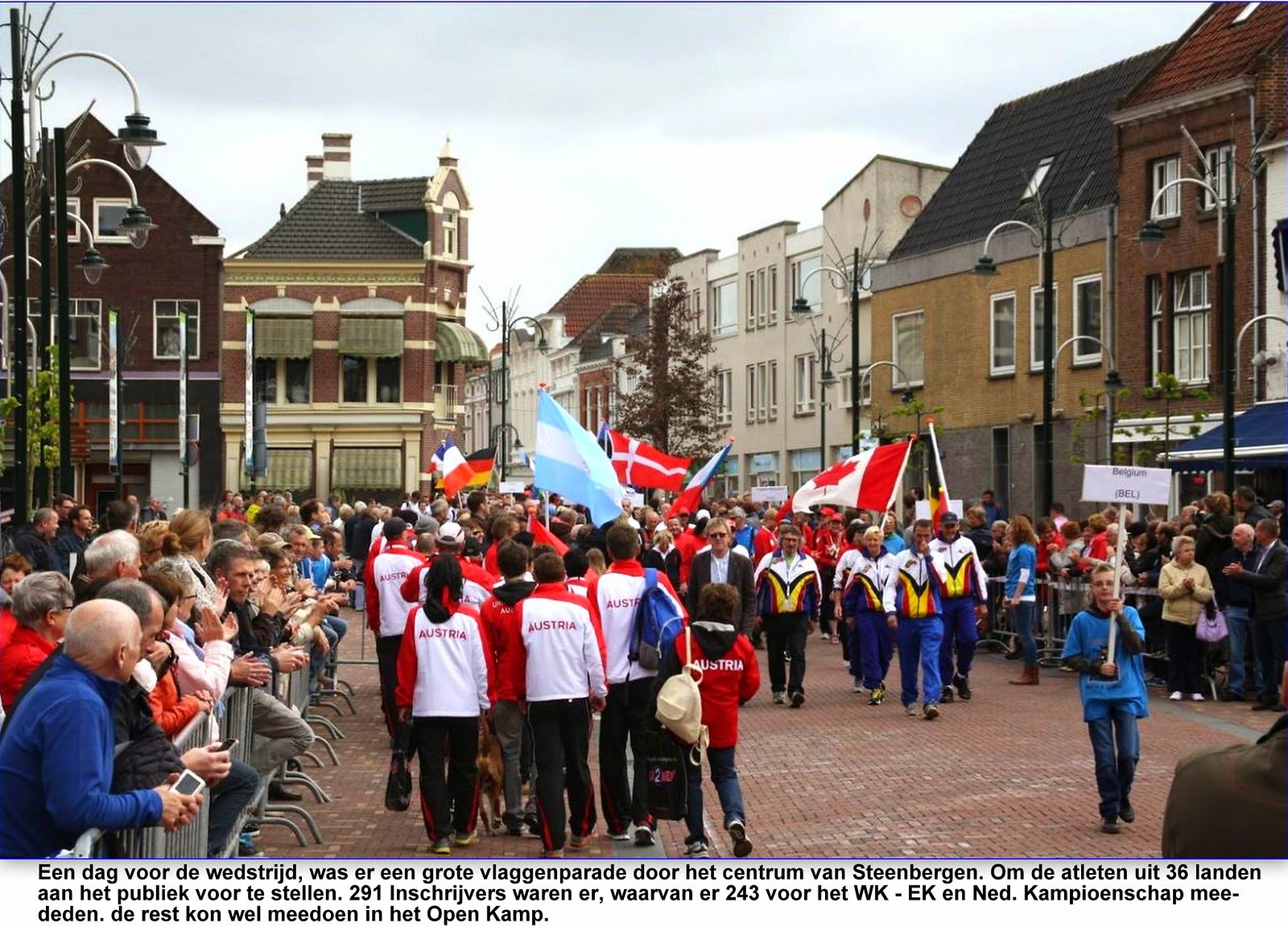The photograph captures a bustling parade taking place on a red brick street in a picturesque, old European-style town under an overcast sky. Crowds of bystanders, held back by metal barricades, line both sides of the street, eagerly watching the procession. Among the parade participants are various groups holding flags from different countries, prominently featuring those of Canada, Austria, and Germany. One noticeable group wears striking red and white jackets with "Austria" emblazoned on the back. Another group, heading towards the camera, is clad in colorful tracksuits of white, blue, yellow, and red, with some members donning black pants. The town showcases a mix of architectural styles, with brown, reddish brick, and white buildings, all adorned with sloping black roofs. Old-style streetlights dot the scene, enhancing the vintage atmosphere. Additionally, a blue outline frames the image, with text at the bottom in a foreign language reading "Yindagbor." Overall, the image vividly depicts a multicultural parade flowing through a charming, historic town, encapsulating a blend of traditional architecture and vibrant, international festivity.